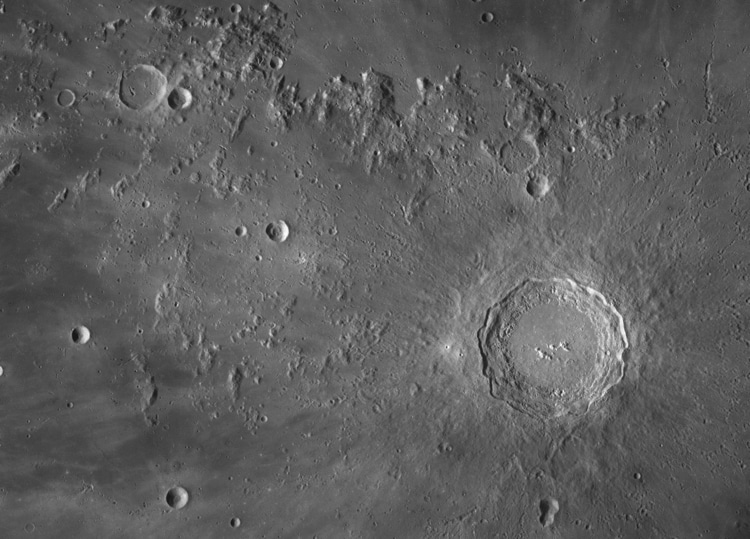The image depicts a black and white close-up photograph of the moon's rugged surface, likely captured through a telescope. Dominating the right side of the image is a large, dome-like crater with grooves on top resembling a cat, flanked by shapes reminiscent of flying birds. This crater is surrounded by thin lines radiating outward, suggesting ancient asteroid impacts and visible shockwave trails. Above this main feature are two smaller craters with mounds of accumulated moon dust. Scattered across the left half of the image are several smaller craters and dots, further indicating a history of numerous impacts. The surface texture is notably uneven, with varying shades of gray highlighting the moon's intricate topography.